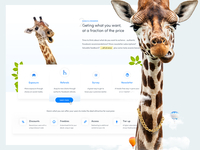The web page features a predominantly light gray background. On the right side of the page, there's an image of a giraffe with distinctive details: it has a white interior, gray-edged ears, a brown top of the head, black eyelids, a brown nose, and a checkered neck combining dark gray and off-white squares. To the left of this giraffe is another giraffe head and neck, similarly detailed. Toward the right of the page, there is some black text, followed by blue text at the top, transitioning to black and then lighter gray fonts. There is also a white box featuring blue text above gray text. A blue circle with white lettering is located centrally. Further down, there's a line of gray text followed by additional lines of gray text interspersed with white squares and small blue images. The content concludes with a line of lowercase gray text.